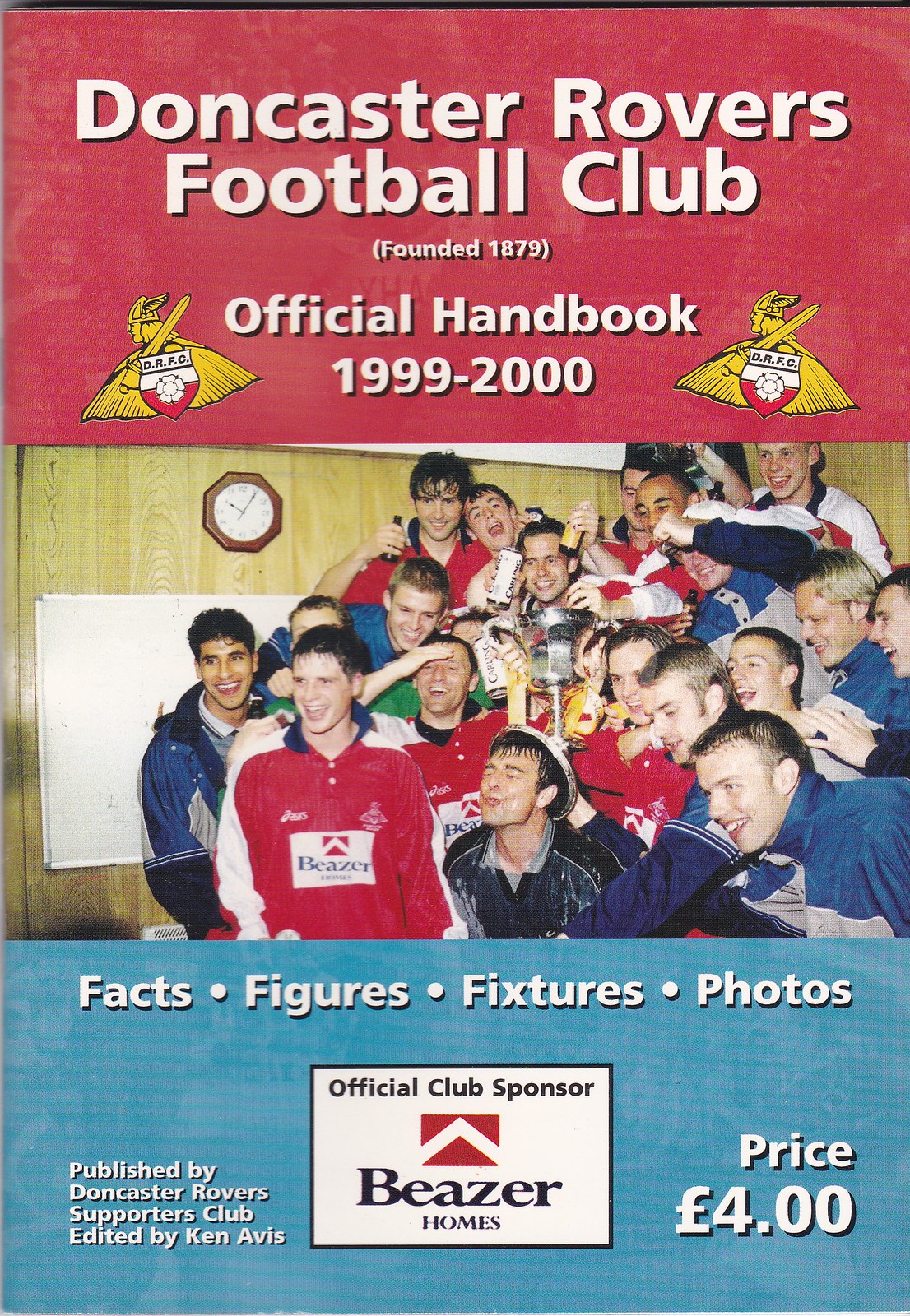The image features a vintage 1999-2000 official handbook of the Doncaster Rovers Football Club, founded in 1879. The top section of the cover is red, adorned with white text, stating "Doncaster Rovers Football Club, Founded 1879, Official Handbook 1999-2000." Flanking this text are two club logos featuring a knight in a winged helmet, wielding a sword, and draped in a cape, with a black, white, and red shield bearing the initials BRFC in front. Below this, a photograph captures a jubilant soccer team or fan group holding a silver trophy, celebrating with evident enthusiasm. Beneath the photograph, a blue box contains the white text "FACTS, FIGURES, FIXTURES, PHOTOS." At the bottom left corner, the text reads "Published by Doncaster Rovers Supporters Club, Edited by Ken Avis." The center-bottom section denotes "Official Club Sponsor, Beezer Homes," while the lower right corner lists the price as £4 or €4.